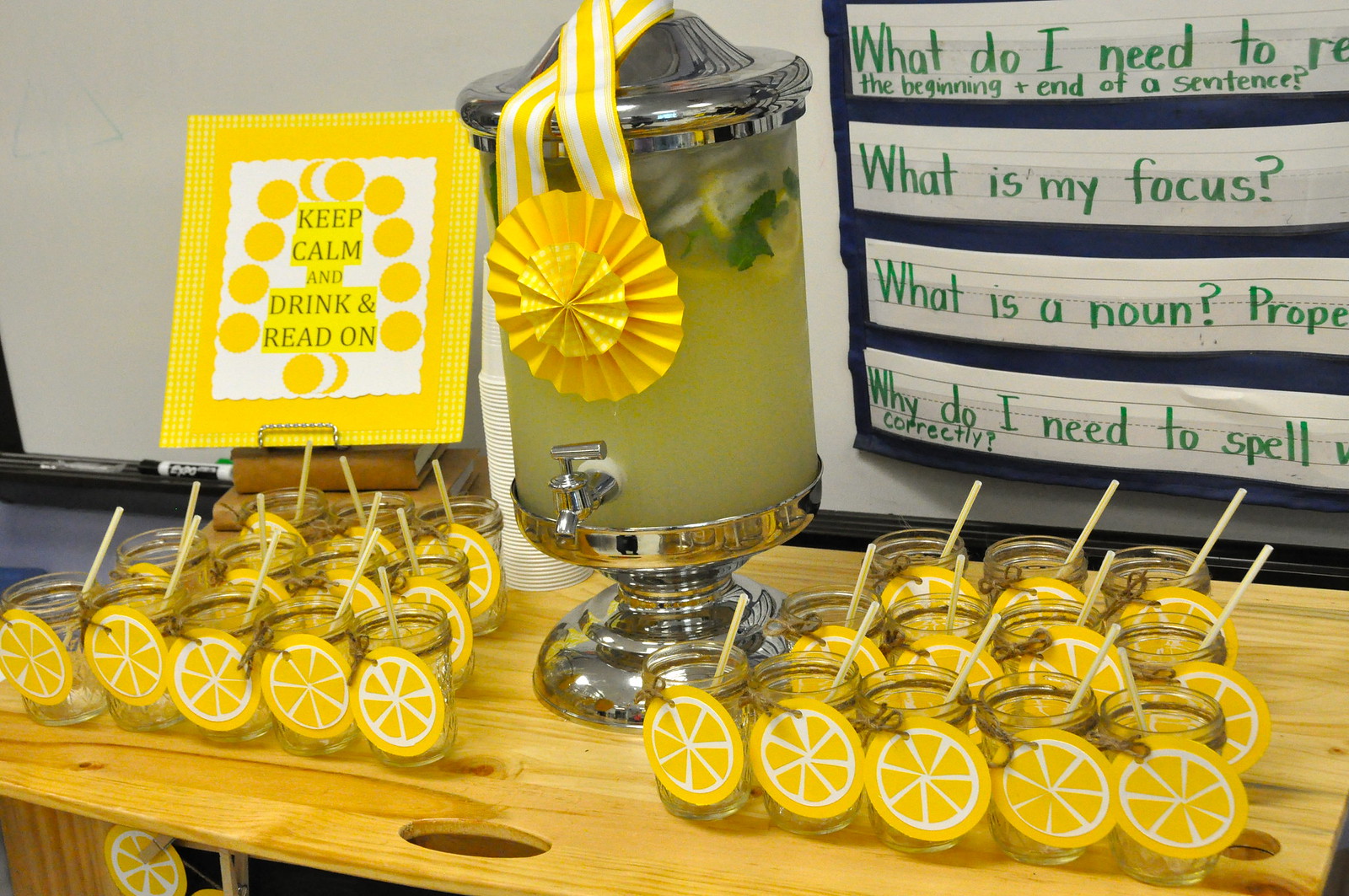This photograph captures a vibrant and inviting lemonade stand, set up on a wooden table. Dominating the center of the scene is a large glass container filled to the brim with refreshing, ice-cold lemonade, accentuated with a gleaming silver base and a practical silver faucet near its bottom for easy pouring. The lemonade, a striking yellow hue, immediately draws the eye.

Surrounding this central jar are numerous clear glass mason jars, each adorned with a cheerful lemon slice sticker and containing a straw, ready for serving. There are probably about 20 to 25 jars, organized neatly for ease of access. To the left of the setup, there's a bright yellow sign that reads, "Keep Calm and Drink and Read On," adding a touch of whimsy and context to the scene.

On the right side, a board is visible with educational prompts and questions such as, "What do I need to read?", "What is my focus?", "What is a noun?", and "Why do I need to spell correctly?", suggesting that this lemonade stand might be part of an educational event or activity. The setup marries refreshment and learning in a visually appealing and functional manner.